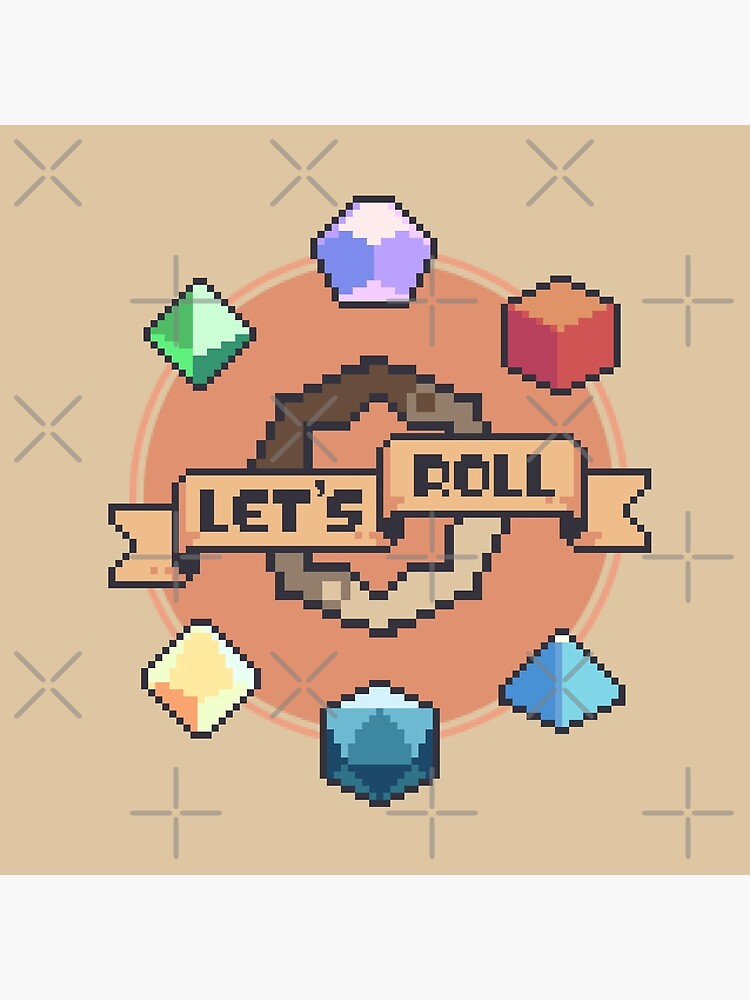This small square digital clip art features an orange circle at its center with a thin orange frame around it, all set against a tan background interspersed with gray X's and plus signs watermark. Inside the circle, there is a pixelated banner in light orange spanning across it, bearing the words "Let's roll" in black. Surrounding the banner within the orange circle are six pixelated, jewel-like structures, with three positioned on the top and three on the bottom. The jewels exhibit varying colors: at the top are emerald green, lavender, and a brown square; at the bottom are peach, dark blue, and light blue. Additionally, there are shapes resembling D&D dice, including a cube and a pyramid. The pixelated elements and watermark maintain the image's distinct, authorized appearance, while a thick white border frames the entire composition, enhancing its defined structure.